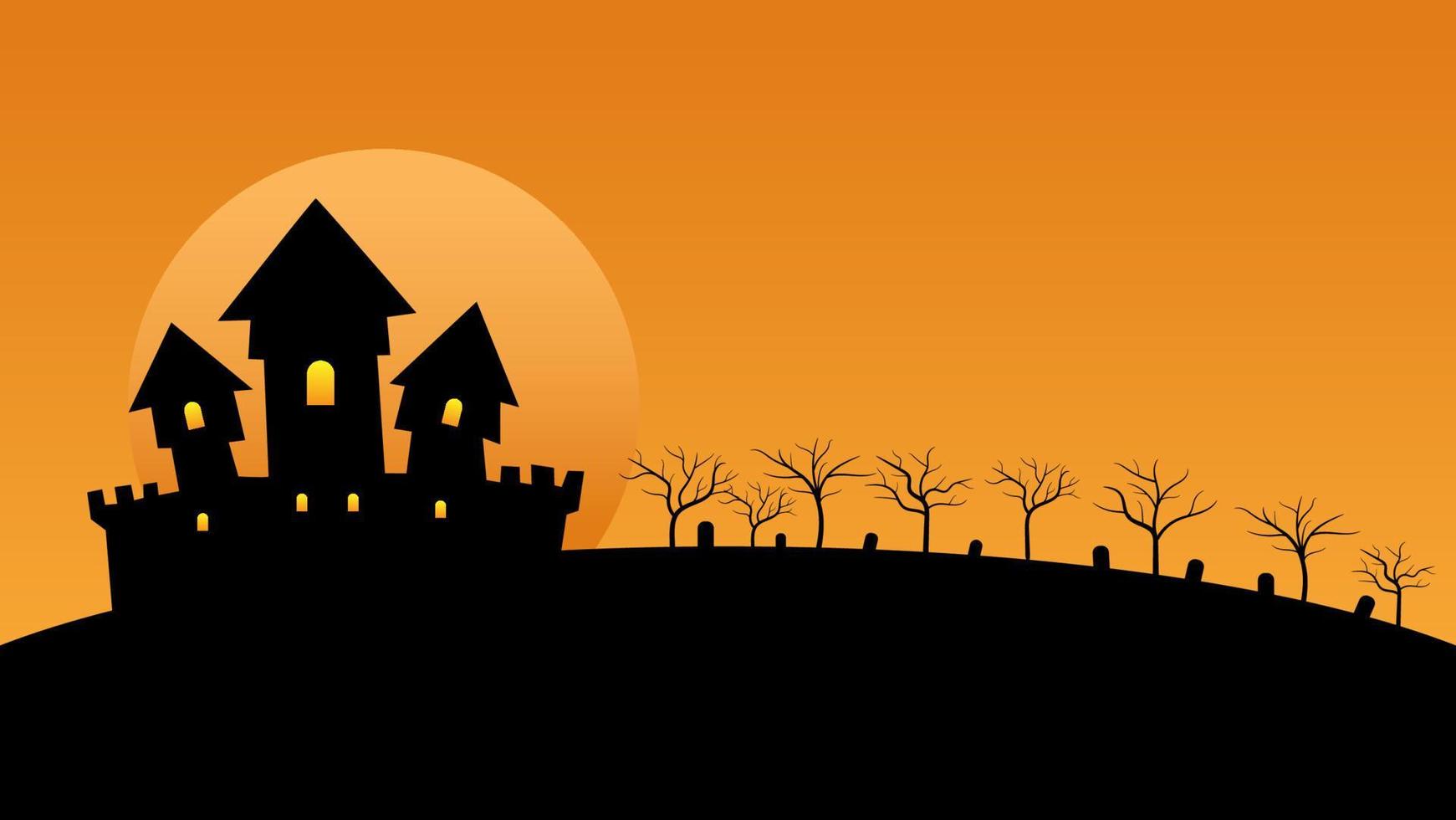This Halloween-themed illustration showcases a surreal, stylized scene set against a bright orange sky. Dominating the left side of the image is a silhouetted black castle, featuring three distinct towers with the central one being the tallest, adorned with parapet-like structures. Glowing yellow-orange light emanates from the castle’s windows, adding a spooky yet inviting touch. Behind the castle, a lighter orange moon rises, adding to the eerie ambiance.

The horizon below is painted a solid, deep black, curving gently upward. To the right, a series of bare, leafless trees also stand silhouetted against the orange sky. Nestled among these trees are roughly nine dark gravestones, contributing to the scene's haunting atmosphere. The entire composition is devoid of text, focusing purely on its vivid, cartoonish portrayal of a classic, spooky Halloween scape.